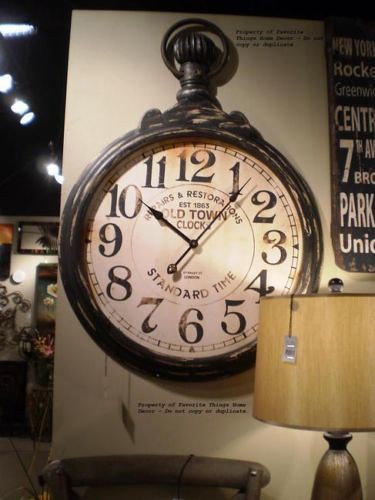The image depicts an intricately detailed, photorealistic poster of a large, black, old-fashioned pocket watch with a white clock face. The pocket watch, with its long minute and second hands and large, ornate black numbers, dominates the scene. The watch face reads, "Repairs and Restoration, Established 1863, Old Town Clocks, Standard Time." It is shown in sharp contrast against an off-white background. In the foreground, there is a wooden table lamp with a tan lampshade, which has a price tag hanging from it, indicating that the setting is a store. The setting appears to be a gift shop, antique shop, or possibly a furniture showroom filled with various items, including more lamps and art objects visible in the background. The overarching ambiance is of a warehouse or industrial-style space, reinforcing the notion that everything displayed, including the heavily advertised pocket watch poster, is for sale.